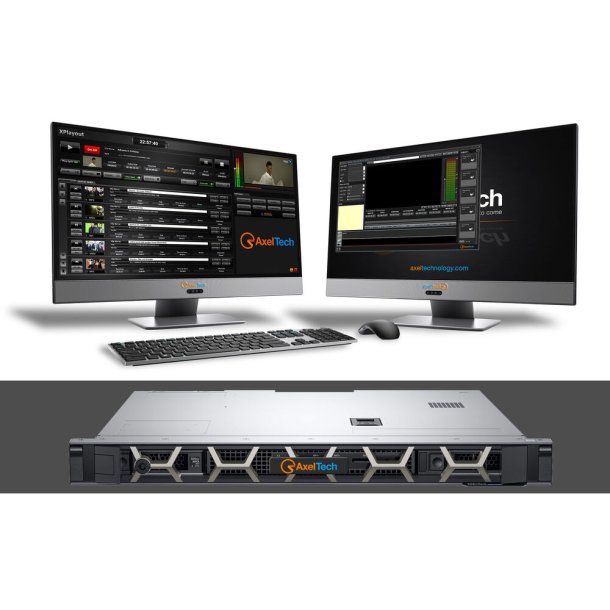The image is a professional, color photograph showcasing a sleek, modern technology setup. The main focus comprises two large, flat-screen desktop monitors positioned on a minimalist, clean podium. The left monitor features a video of a man in the top right corner, with various media websites open against a black screen. The right monitor displays a web elementary streaming interface. In front of the monitors is a compact wireless keyboard with black keys on a silver background, accompanied by an ergonomically designed cordless mouse in dark gray. Below the monitors, a smaller close-up photograph captures a sophisticated, grey digital disk storage unit adorned with the brand name "AxelTech" in striking orange and blue text. The entire setup exudes a futuristic and uncluttered ambiance, further emphasized by the absence of visible wires against the white background.